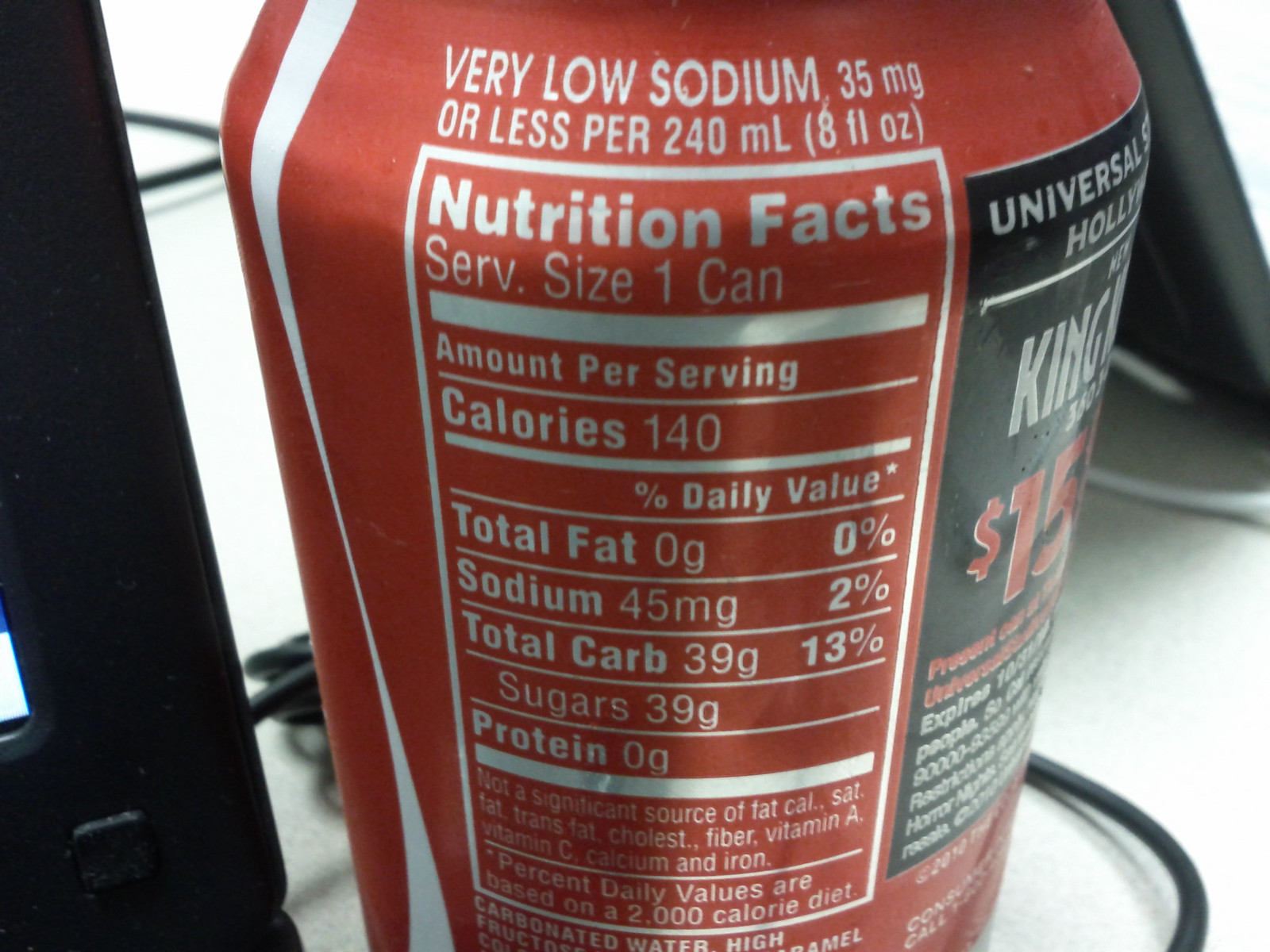The image depicts a close-up of the back of a red Coca-Cola can adorned with a white stripe, reminiscent of the iconic Coca-Cola design. The visible nutrition facts label indicates the following: very low sodium, 35 milligrams or less per 240 milliliters (8 fluid ounces); serving size of one can; 140 calories per serving; 0 grams of total fat; 45 milligrams of sodium; 39 grams of total carbohydrates, comprising 13% of the daily value; 39 grams of sugars; and 0 grams of protein. Some ingredients are partially visible, mentioning carbonated water and high fructose, but the list is cut off. Additionally, to the left, there is a black square that seems to be a promotional section, possibly for a contest related to Universal Studios Hollywood, showing partial text including the word "king" and the number "15". The can is placed on a white table amidst black and white cords and appears to be near a screen.